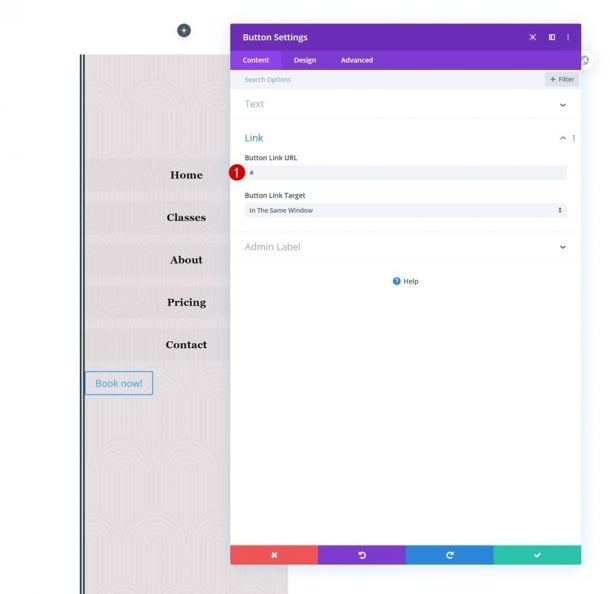This image is a detailed screenshot of a user interface with a sidebar and a settings panel. On the left portion of the image, the sidebar has a lavender-colored background with a list of items in black font. The items listed include "Home," "Classes," "About," "Pricing," and "Contact." Below these items, there is a "Book Now!" button in blue font, outlined with a blue rectangle.

The majority of the image is occupied by a vertical settings panel with a white background. The top border of this panel is purple, with "Button Settings" written in white font. Below this header, there is a three-item menu labeled "Content," "Design," and "Advanced," all written in white.

In the main section of the settings panel, under the "Search Options" label, there is a "Text" section featuring a gray downward-pointing arrow indicating a dropdown menu. Below it, the "Link" section includes an entry labeled "Button Link URL" accompanied by a red circle with a white number "1." Another gray rectangle below this is labeled "Button Link Target," with "In the Same Window" written inside it. Further down, the "Admin Label" section also includes a dropdown arrow.

At the bottom of the panel, there is a small gray "Help" link with a blue circle and a white question mark next to it. The very bottom of the settings panel features four colored blocks (red, purple, blue, and green), each containing a white symbol: an "X," a left-pointing arrow, a right-pointing arrow, and a checkmark, respectively.